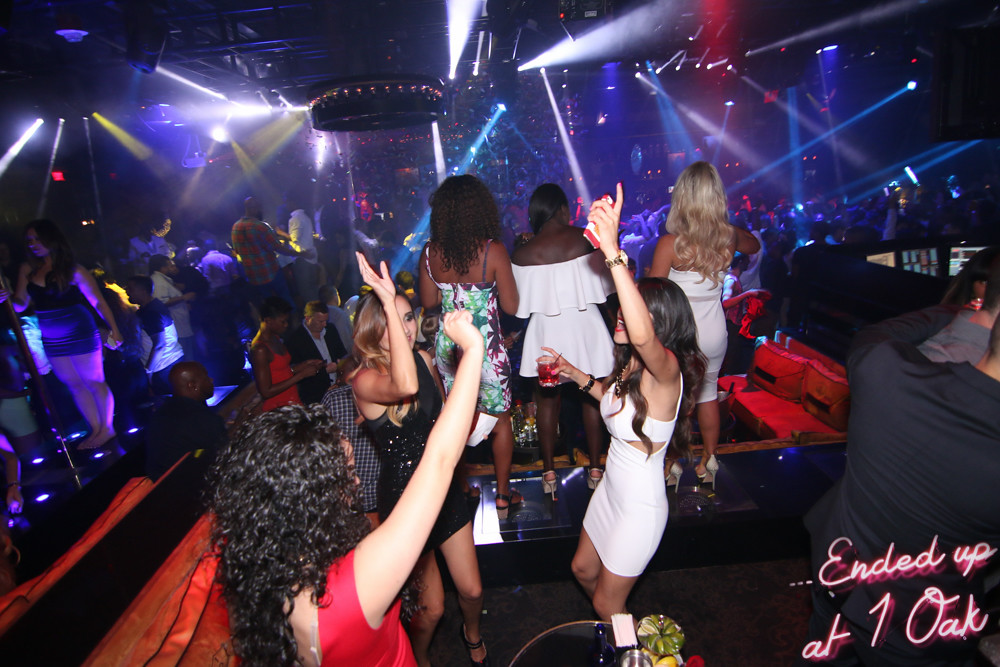This lively snapshot captures the vibrant atmosphere of a nightclub, "One Oak," filled with colorful lights and a dynamic crowd. At the center of the image, prominently on a glass dance floor, are three women raising their drinks in a celebratory toast, each with one hand held high. 

The first woman stands out in a tight, short white tank dress, sporting a red cocktail in her right hand, a watch, and a cellphone in her left. The second woman, with long blonde hair, dons an even shorter black dress paired with black heels, emphasizing her spirited presence. The third woman, with long black hair, is dressed in a red outfit cropped at her chest, lending a touch of mystery to her ensemble. 

Surrounding them are various other club-goers, engaged in dancing and mingling, illuminated by an array of spotlights and strobe lights in hues of blue, white, yellow, and red, giving the scene a pulsating, energetic vibe. The photo also captures the text "ended up at One Oak" at the bottom right corner, indicating the venue. 

In the background, a DJ is seen spinning tracks, setting the musical tone for the evening, while the VIP area, marked by an orange velvet couch, adds an exclusive touch to the scene. Adjacent to the dance floor and to the left, a bustling bar area further adds to the ambiance, with patrons enjoying their drinks. The entire setting suggests an indoor, nocturnal environment, epitomizing the excitement and social buzz of a night out.